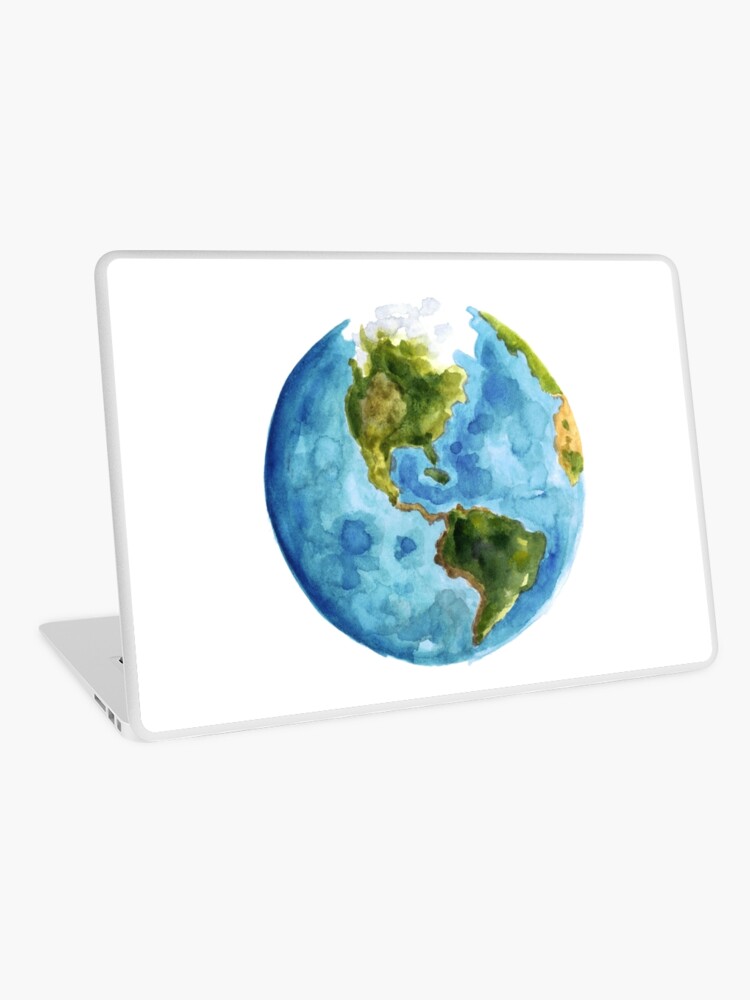The image is a computer-rendered graphic of a modern, flat-screen laptop with a sleek design. The laptop is predominantly gray and white, and it's open with the screen facing away from the viewer, exposing small ports on the left side including an ethernet and SD card slot. The entire scene is set against a white background. On the back of the laptop screen, there is a stylized, watercolor-like artwork of the Earth featuring North and South America, with Greenland shown at the top, partially covered by ice. The oceans around the continents are depicted in a spotty bluish-turquoise color, and there's a hint of green and yellow near the top right of the globe. The laptop appears to have a white cover, giving a clean, polished look to the device.